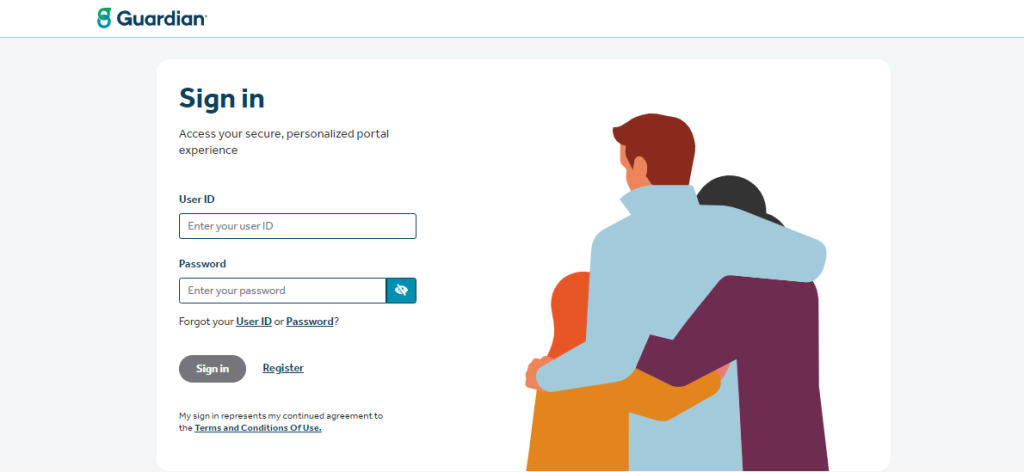This is a screenshot of a web page belonging to "Guardian." The webpage's background is predominantly white, featuring a large, rectangular, very light blue box. Within this large box, there is a smaller white box containing the essential information.

At the top, the title "Guardian" appears, accompanied by a small green and blue symbol. Below it, in large blue letters, is the heading "Sign In." Underneath the heading, there is a text stating, "Access your secure personalized portal experience."

The first input field is labeled "User ID" in blue, with a placeholder text inside the box prompting the user to "Enter your user ID." Below this, a second rectangular input field labeled "Password" in blue invites users to "Enter your password." Inside this field is a small blue icon featuring an eye with a line through it, allowing users to reveal their password if clicked.

Directly beneath these fields, there is a text link reading "Forgot your User ID or Password?" Below this, there are two buttons: a blue "Sign In" button and a grey "Register" button. Following these buttons, there's a disclaimer: "My sign in represents my continued agreement to the Terms and Conditions of Use."

To the right of the sign-in form is an illustrative drawing depicting three people - a man hugging a woman and a child - adding a personal touch to the otherwise business-like webpage.